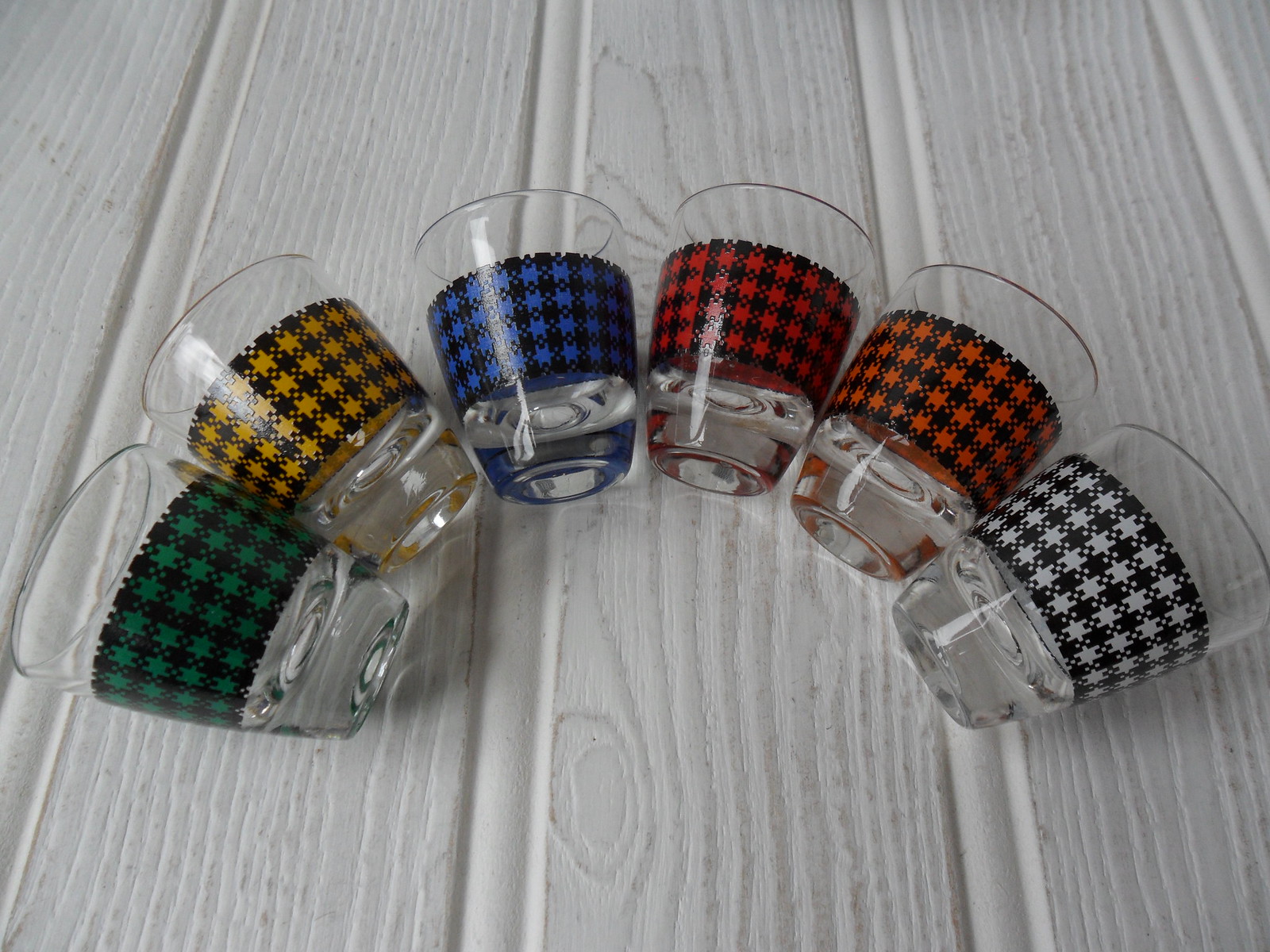The photograph showcases a white wooden tabletop, where the wood grain is visible through the white paint. Arranged in an arch on the tabletop are six shot glasses, each adorned with a distinct houndstooth pattern. The glasses are positioned side by side, creating a rainbow-like semicircle. Each glass shares a black element in its houndstooth design but varies in its secondary color: green and black, yellow and black, blue and black, red and black, orange and black, and finally, black and white. The intricate houndstooth patterns form thick bands that wrap around the body of each glass, emphasizing their uniform yet colorful variation.